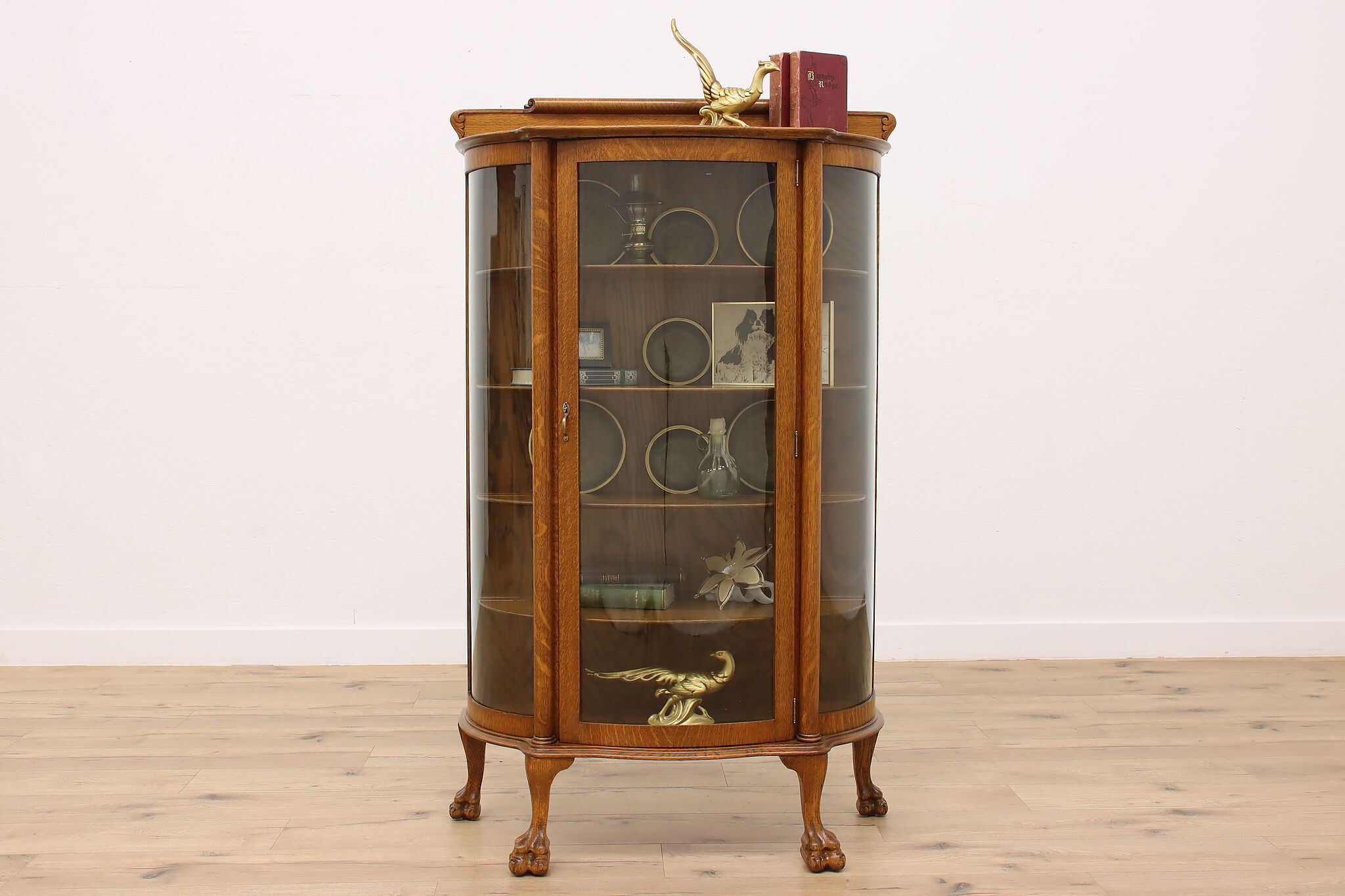This detailed image features an elegant curio cabinet crafted from dark tan wood, standing securely on four intricately carved legs resembling animal feet. The cabinet boasts three glass panels and three interior shelves, encapsulated by circular sides, with a door on its front. Atop the cabinet rests a gold bird ornament and two vintage red books, all against a background of a light wood floor and a slightly off-white wall.

Inside the cabinet, the top shelf displays three gold circular objects and an oil lamp. The second shelf holds a book lying flat, topped by a photo frame and another gold circle, alongside a portrait of a dog. The third shelf contains three additional gold circles and a candle in a jar. The bottom shelf houses two books, a floral decoration, and another gold bird ornament. The entire scene is meticulously composed, likely captured using a tripod for a perfectly straight angle.